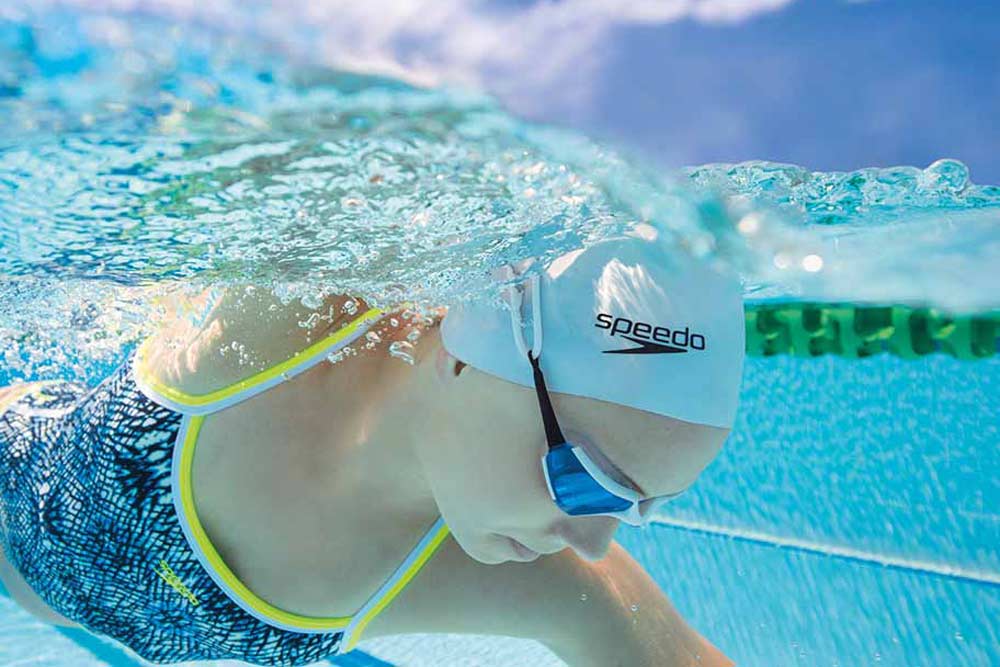This underwater photograph captures a close-up of a female swimmer performing a front stroke. The water is crystal-clear blue, creating a serene and vivid backdrop. The swimmer, a white female, is seen in a blue one-piece Speedo swimsuit with distinctive yellow trim on the bikini top. She also sports a white Speedo swimming cap with a black logo and white goggles with black trim and purplish lenses that obscure her eyes. Her face is positioned downward as she swims, emphasizing her focus and form. The image also briefly captures the edge of the pool with green lane markers and bubbles near the back of her head, indicating her movement through the water. Above the water, the sky peeks through with clear blue hues and scattered white clouds, although it remains slightly blurry compared to the crisp underwater clarity.